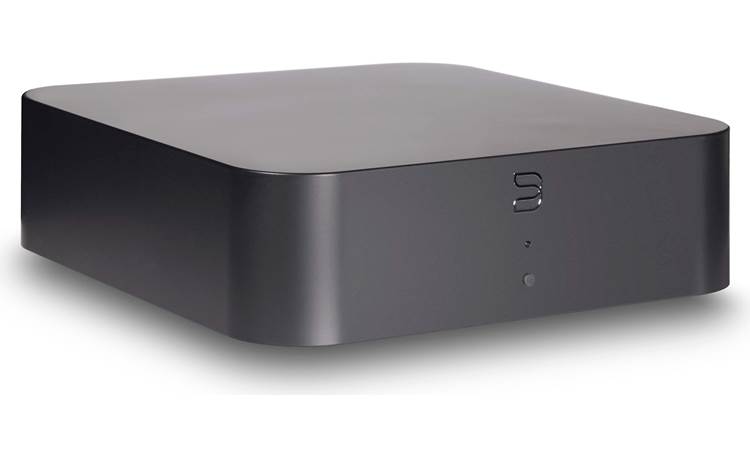The image features a small black plastic box with rounded corners, approximately an inch high and three inches wide, set against a white background. The box has a flat top and a design on the front, which includes a unique logo resembling a sideways U-shape crossed at the bottom. Beneath the logo are two small circles, possibly indicating functionality or status lights. The front also features a small white or clear knob that may light up when the device is in use. This item is suspected to be some sort of tech equipment, possibly a TV streaming player or router, reflecting its sleek and modern design. There is no text present in the image, and the focus remains solely on the black box with its intriguing geometric details.